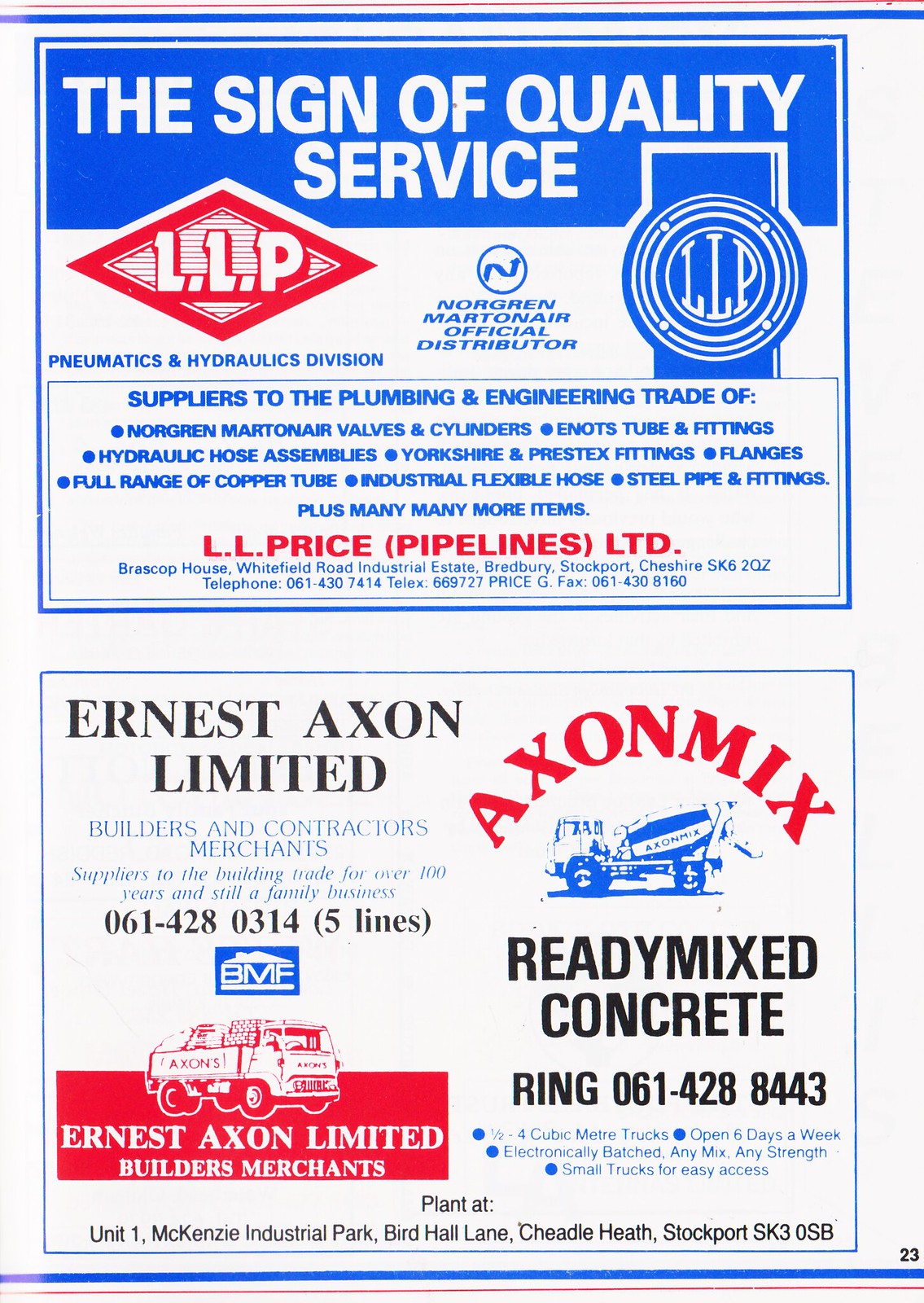The image is a page from a magazine featuring two advertisements, both prominent in blue and red hues. At the top of the page, the first advertisement showcases "The Sign of Quality Service, LLP," accompanied by a red, diamond-shaped logo with "LLP" encircled. This advertisement further identifies itself as the official distributor for Norgreen Martinaire's Pneumatics and Hydraulics Division, supplying various products such as valves, cylinders, E-Nuts tube and fittings, hydraulic hose assemblies, Yorkshire and Prestex fittings, flanges, and a full range of copper tubes, industrial flexible hoses, and steel pipes. The supplier's details, including "LL Price, Pipelines Ltd, Brasco Pals, Whitefield Road Industrial Estate, Bradbury, Stockport, Cheshire, SK6 2QZ," and contact numbers can also be found. 

The second advertisement at the bottom highlights "Ernest Axon Limited," featuring blue and red branding elements, including illustrations of a cement dump truck and a hauling truck. It notes the company’s heritage as builders and contractors' merchants, serving the building trade for over 100 years and remains a family business. This section also promotes "Axon Mix," shown in red letters above a blue drawing of a cement mixer, offering ready-mixed concrete in varying quantities, open six days a week, with convenient mix variations and small trucks for easy access. Contact details and location information, such as "Plant at Unit 1 Mackenzie Industrial Park, Birdhole Lane, Cheadle Heath, Stockport, SK3 0SB," are provided, along with phone numbers for further inquiries. The page number "23" is noted at the bottom right corner.